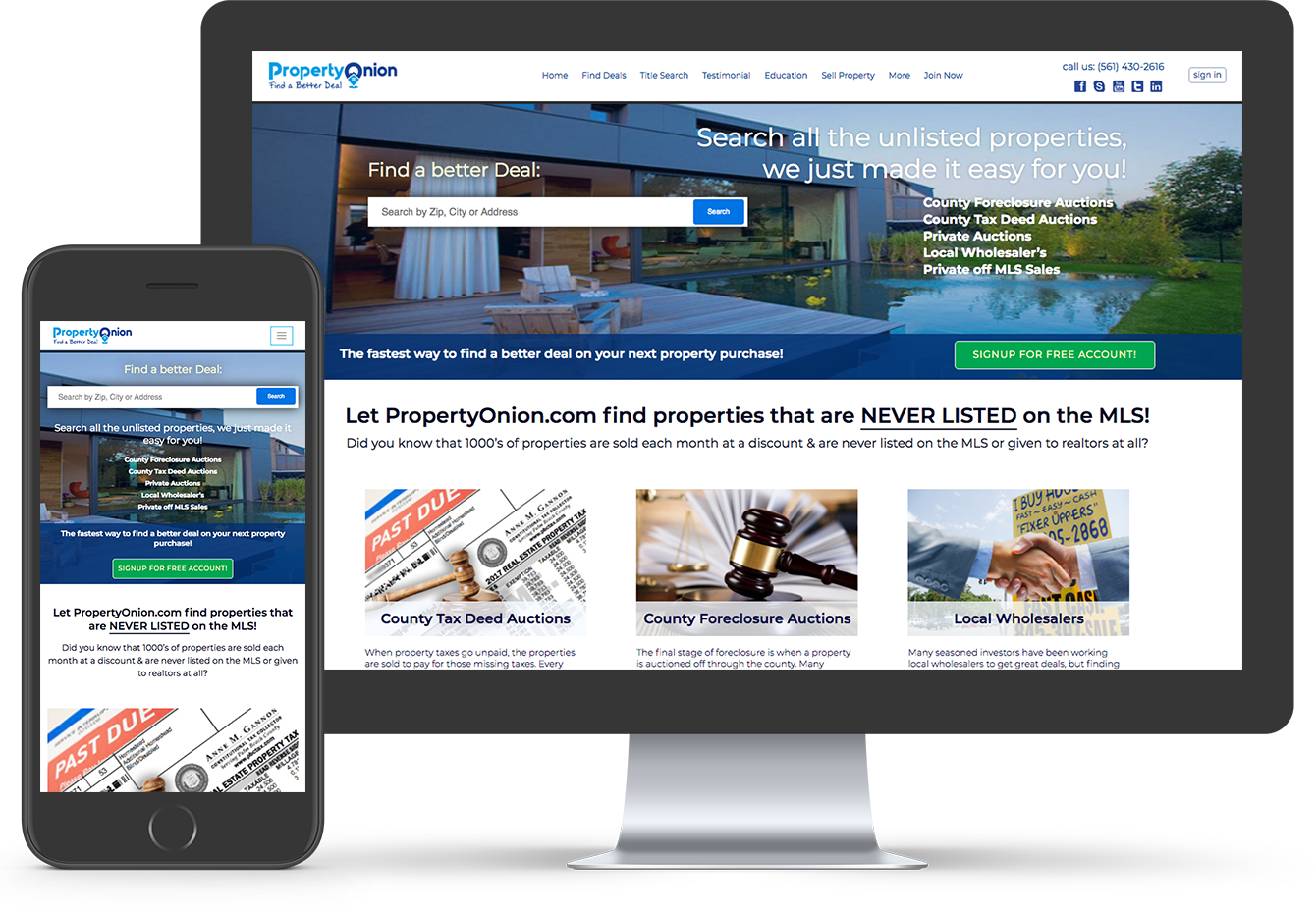This image captioned:

"A promotional image for PropertyOnion.com, a website dedicated to helping users find better deals on real estate. Property Onion specializes in unlisted properties, county foreclosure auctions, county tax deed auctions, private auctions, local wholesales, and private off-MLS sales. The site features a search bar where users can search for properties by city, state, or address, similar to Zillow. The key selling point is access to exclusive listings that are not available on the Multiple Listing Service (MLS). The advertisement highlights that an account is necessary to access these benefits, encouraging potential users to sign up for a membership. Additionally, the platform offers both an app for mobile devices and a website for desktop use, ensuring convenient access to these exclusive real estate deals."